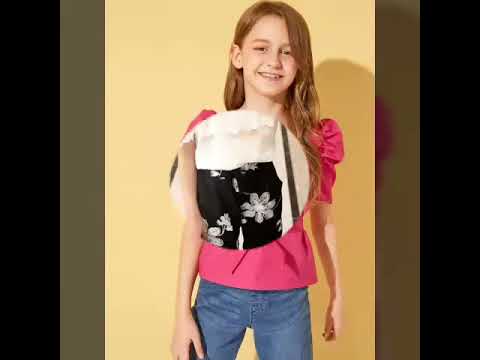A young girl, approximately 8 to 10 years old, stands smiling against a yellow background adorned with black and brown stripes on either side. She has long reddish-brown hair, with the right side tucked behind her ear, and wears a pink shirt with poofy sleeves alongside blue denim jeans. The image appears slightly unusual as her arms seem to be different lengths, hinting at possible AI generation or photoshopping. Superimposed over her chest is a circle depicting another outfit – black pants with white flower patterns and a white top, which might be part of a clothing advertisement. Surrounding the central picture are alternating borders: thin black rectangles on the far left and right, followed by olive green ones as you move closer to the center. Her shadow is cast on the yellow background, enhancing the layered visual effect of this composite image.